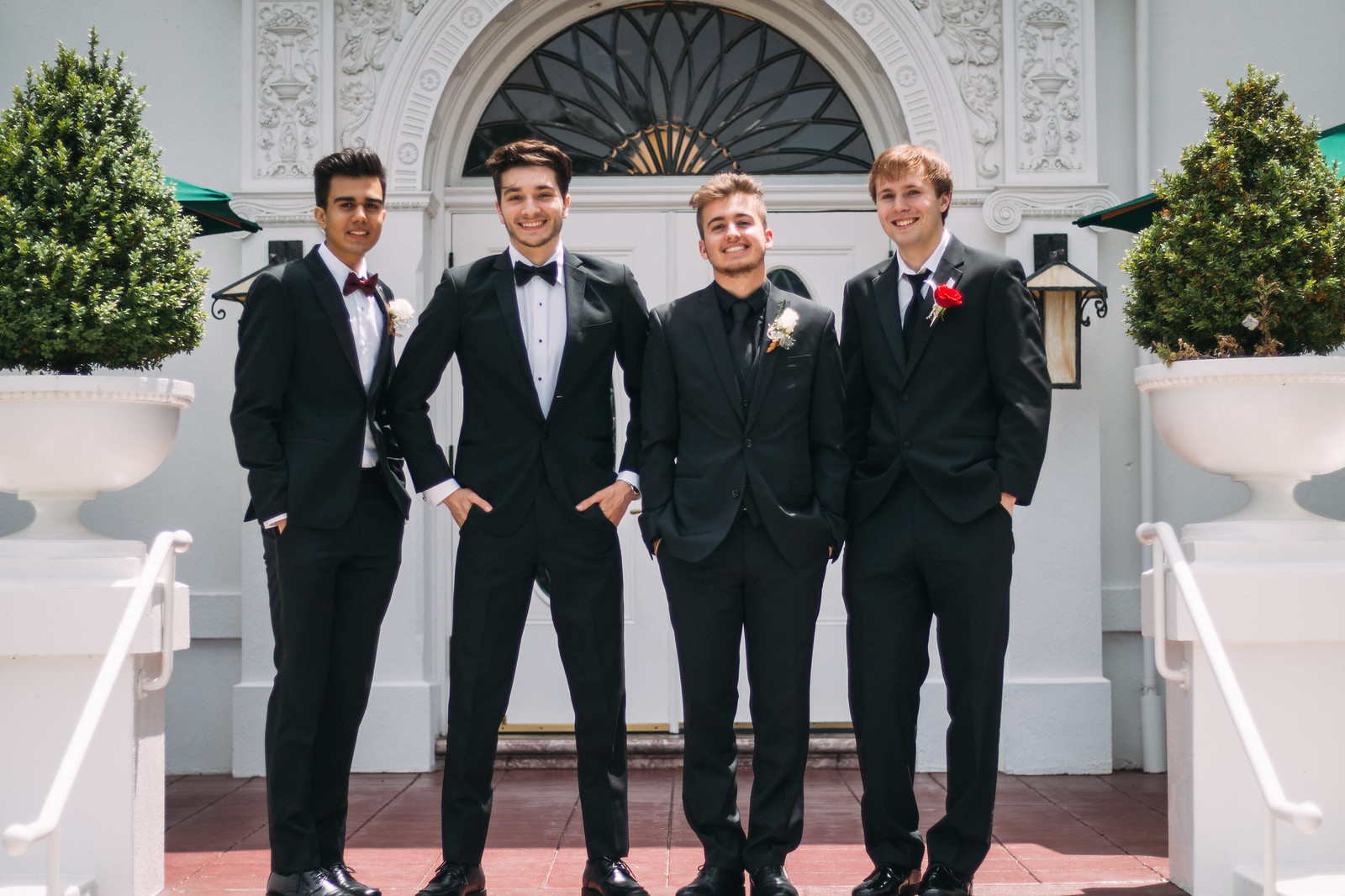This is a detailed photograph of four young men standing in front of a white church, possibly at a wedding. The men are all formally dressed in black suits, with their hands in their pockets, smiling at the camera. From left to right, the first man is in a black suit paired with a white shirt and red bowtie, and he sports a boutonniere on his jacket. The second man, also in a black suit and white shirt, wears a black bowtie but has no flower. The third man stands out with a completely black ensemble - black suit, black shirt, black tie, and a white flower boutonniere on his left lapel. The fourth man, taller than the others, has a black suit, white shirt, long black tie, and red flower boutonniere.

They are positioned on what appears to be a reddish-brick tiled surface. Behind them, the closed double doors of the church are framed by an archway and flanked by two small green shrubs in white planters. Matching white railings can be seen on either side, suggesting the presence of stairs leading up to the entrance, which is marked by a distinct stained glass window above the doors. Two of the men, possibly Hispanic or Asian, are on the left, while the two on the right appear to be Caucasian.